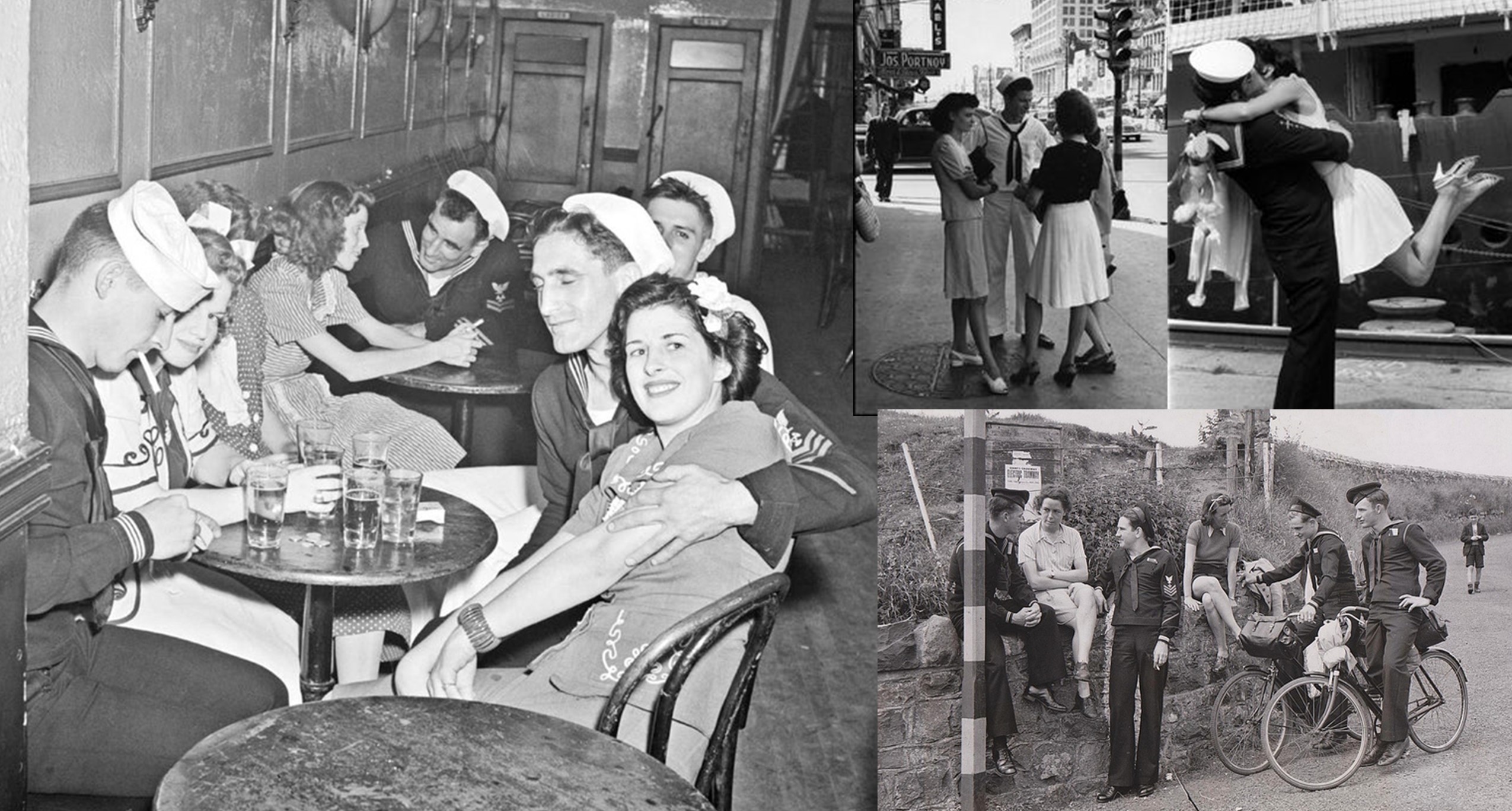This image is a meticulously crafted collage of four vintage black-and-white photos, likely from the 1930s or 1940s, capturing the intimate and joyous moments of Navy men and women during wartime. The largest photo, situated on the left side, shows sailors in their white hats and uniforms sitting at tables with women in what appears to be a restaurant. These tables, adorned with glasses, host multiple couples engaged in lively interaction; one man, eyes closed, embraces a woman while another smokes contentedly beside his companion. In the background, a man is seen speaking to a woman, accentuating the convivial atmosphere.

In the top right corner, there is a heartwarming scene of a sailor in a black uniform with a white hat lifting a woman in a white dress and heels off the ground, presumably kissing her in a joyful embrace. Below this image, another photograph depicts two men on bicycles conversing with a woman seated on a wall. Another woman and man are also engaged in conversation nearby, with the scene set against a hilly outdoor backdrop, adding a picturesque quality to the composition.

Finally, the remaining photo in the top right showcases a man chatting with three women on the street, further emphasizing the social interactions and sense of community among the service members and civilians. Every individual is clad in period-appropriate attire, adding to the nostalgic and historical significance of this poignant collection.